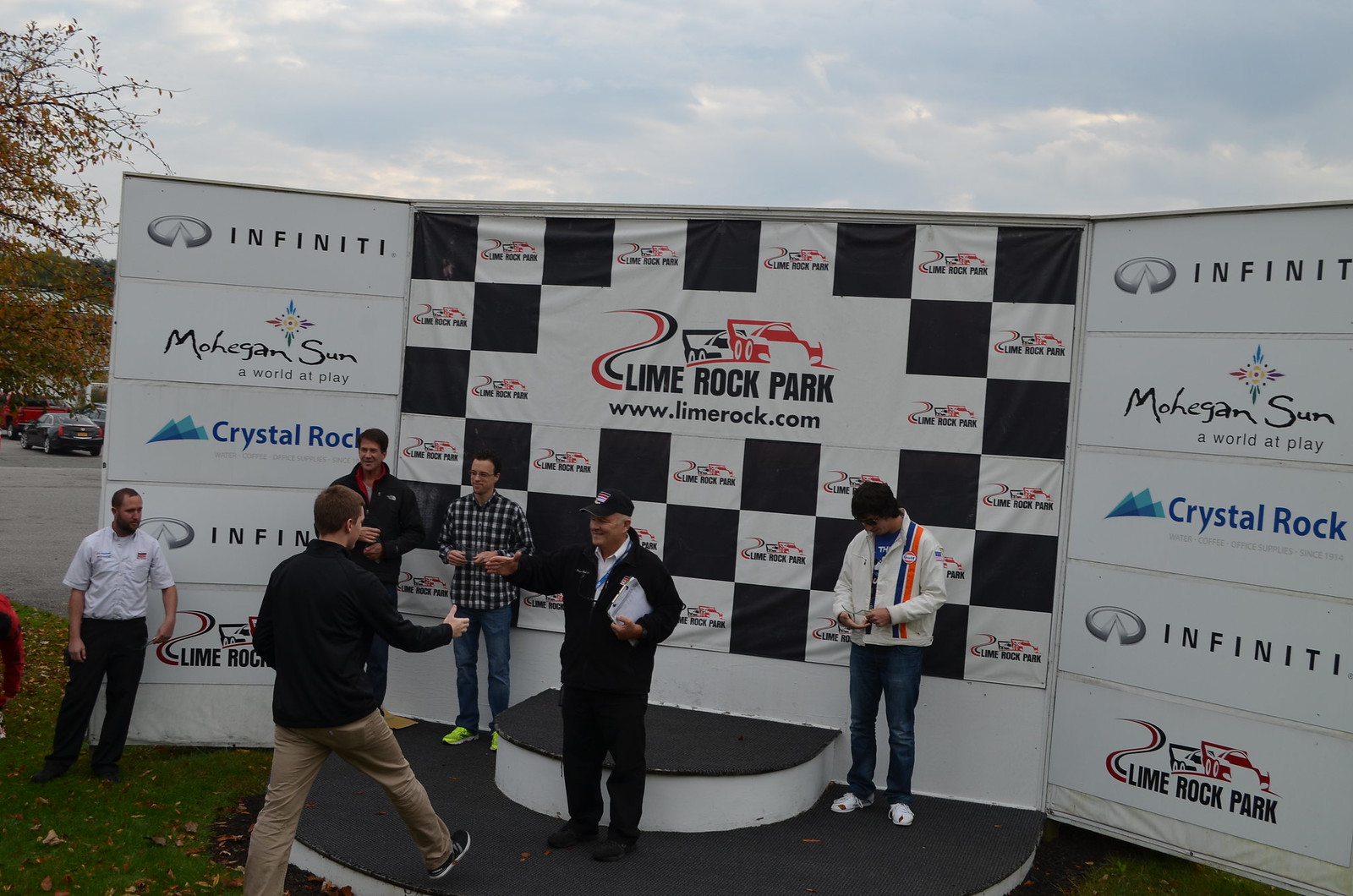The photograph, taken outdoors under a cloudy sky amidst grass and trees, depicts a staged award scenario resembling those seen in sporting events, specifically car racing. The stage, portable and set on grass, serves either for photography or awards. Five white men are present: four standing on the stage and one on the grass nearby. A central figure on the stage, wearing a black jacket, white shirt, black pants, and dark shoes, holding a clipboard in his left arm, is reaching out to shake hands with another man in a black zip-up sweater and tan pants. Surrounding them, other men are positioned on both sides. The background consists of multiple logo boards featuring repeated advertisements for Lime Rock Park, Mohegan Sun, Crystal Rock, and Infinity. Dominating the center is a large, checkered backdrop displaying the Lime Rock Park logo accompanied by the URL, www.limerockpark.com, and illustrations of two racing cars—one black and one red. The scene suggests a post-race award ceremony or photo opportunity.